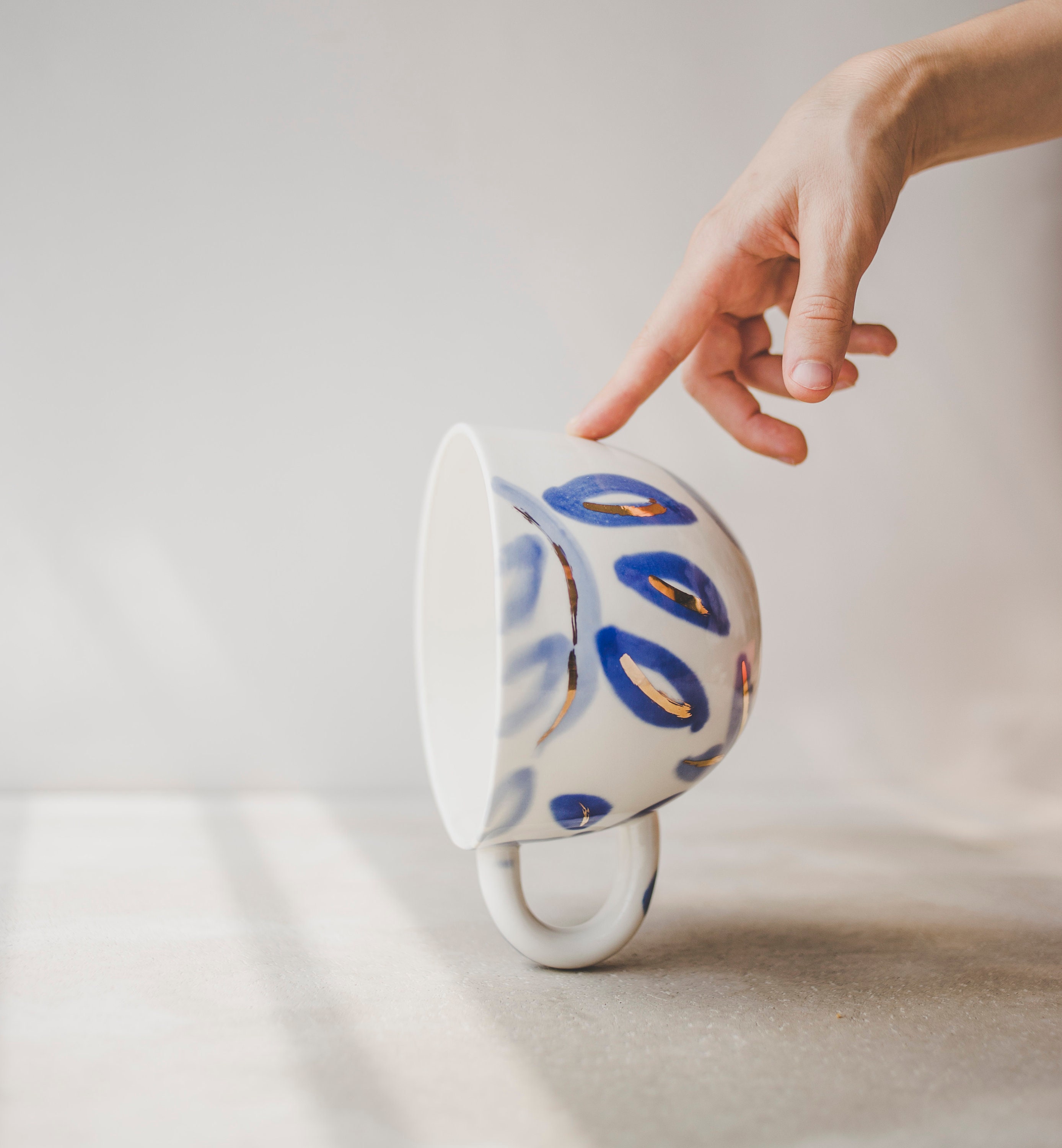This photograph features a teacup artfully balanced on its handle, positioned in the bottom portion of the image. The teacup's open side faces the left side of the frame, while its base is oriented towards the right. The cup is predominantly white with blue oval designs, some of which have gold accents, displaying varying degrees of brightness and fading. Emerging from the top right corner, a light-skinned right hand is seen stabilizing the teacup with an index finger pressing down on its rim to prevent it from toppling. The backdrop consists of a white wall and a surface that appears off-white in some areas, subtly illuminated by light coming from the left side, creating a gradient of light across the scene.